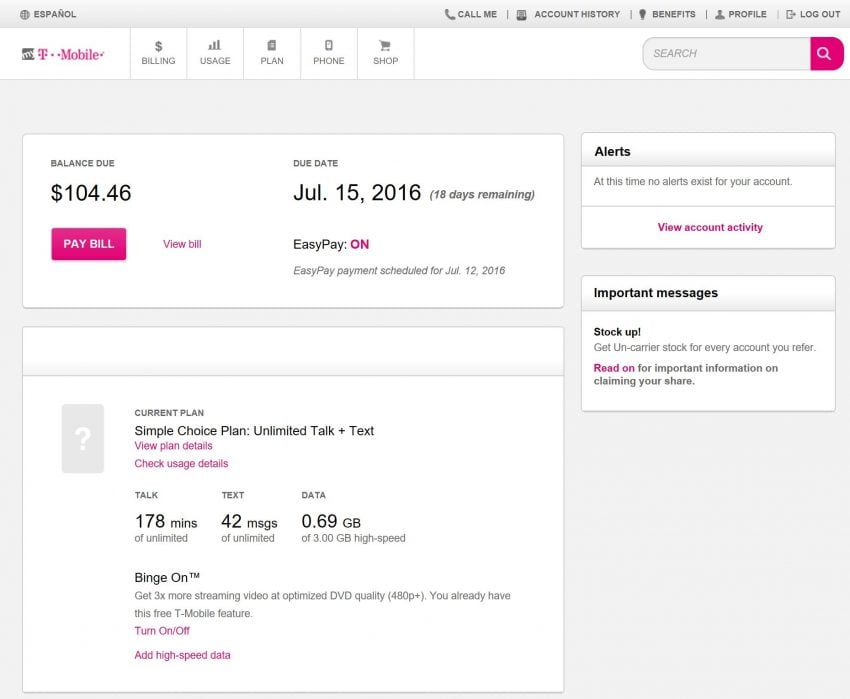Here's a refined and detailed caption for the screenshot based on the given voice description:

---

Screenshot of a T-Mobile customer account summary page on a web browser. The device used to capture the screenshot is unspecified. The web page header includes a dark gray bezel. On the left side, there's a globe icon labeled "Español" for switching the language to Spanish. On the right, icons for "Call Me" and a silhouette for "People" are followed by a "Logout" button symbolized by a square with a right-pointing arrow.

The T-Mobile logo is positioned on the left, with "My" displayed in white within a black square alongside the hot pink "T-Mobile" text. Below the header are several tabs delineated by gray lines: "Billing" with a pass symbol, "Usage" with a graph, "Plan" with a paper icon, "Phone" with a phone illustration, and "Shopping" represented by a shopping cart.

To the right is a rounded gray search bar flanked by a hot pink magnifying glass icon. A dark gray rectangle below displays the balance due, $104.46, with a hot pink "Pay Bill" button and a "View Bill" hyperlink in hot pink. The due date, July 15, 2016, and the time remaining (18 days) are also highlighted. "Easy Pay" status is shown as "On" in hot pink, with the next payment scheduled for July 12, 2016.

A floating rectangle on the right under a gray bezel labeled "Alerts" indicates no existing alerts, with a hot pink "View Account Activity" hyperlink below. Beneath is another dark gray rectangle titled "Important Messages" in bold black text. Inside, a promotional message encourages users to refer accounts for un-carrier stock, with details available via a "Read On" hyperlink.

In the final section, a dark gray square with a white question mark outlines the "Current Plan," labeled as "Simple Choice Plan: Unlimited Talk + Text." There are clickable links for more details such as "View Plan Details" and "Check Users Details" in hot pink. Subsections list usage details: 178 minutes of talk, 42 text messages, and 0.69GB out of 3GB high-speed data used. The plan includes "RingOnTM" for optimized video streaming and data management options, with a hot pink hyperlink for adjusting high-speed data settings.